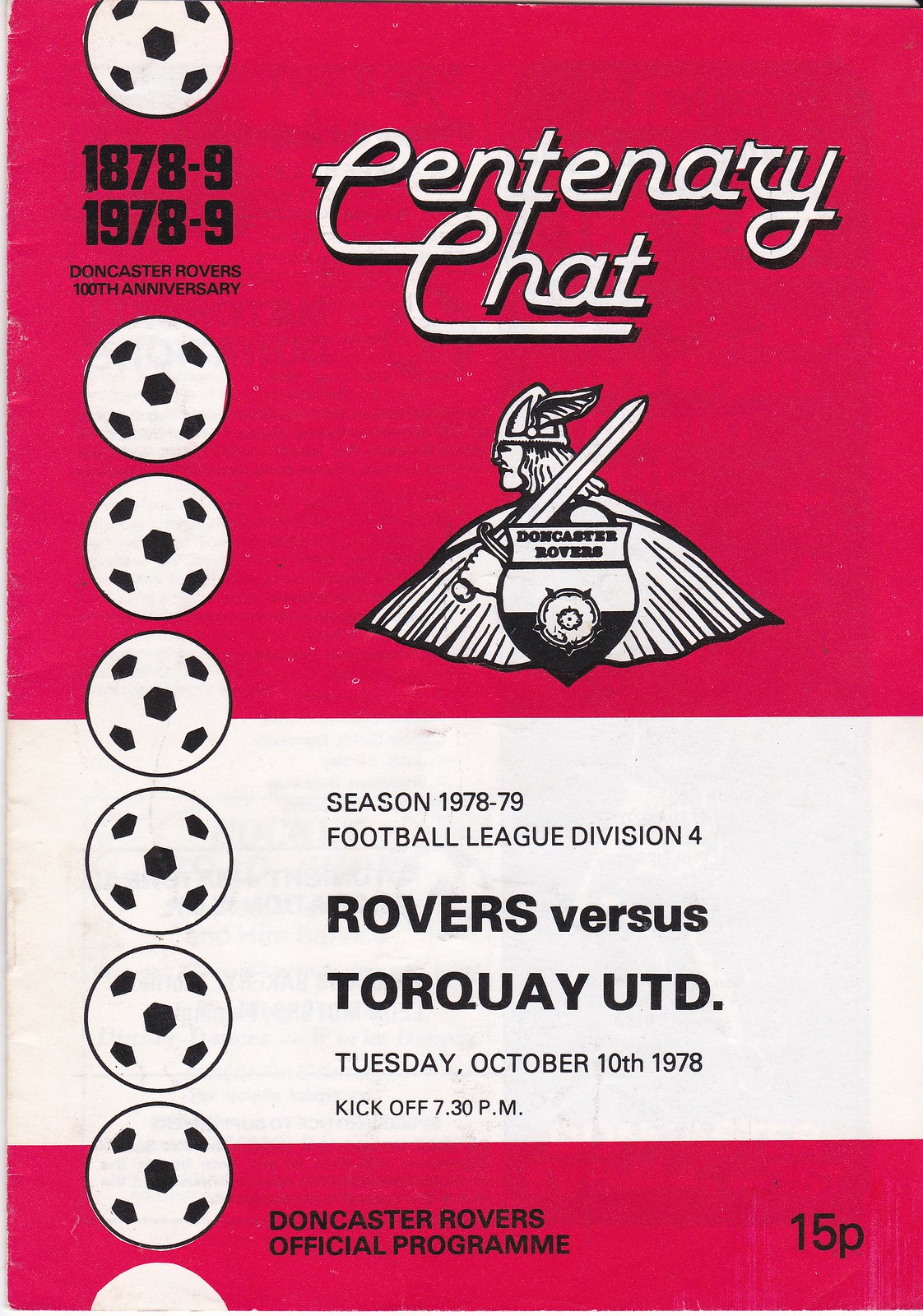This is a vintage program cover from a 1978 soccer match featuring Doncaster Rovers against Torquay United, celebrating the Rovers' 100th anniversary from 1878 to 1978. The design consists of a large red section at the top adorned with seven soccer balls aligned on the left and the title "Centenary Chat." Beneath this header is the Doncaster Rovers emblem, featuring a Viking warrior holding a sword and shield draped in a cape, symbolizing the team's mascot. The middle white portion of the program highlights the event details: "Season 1978-79, Football League Division 4, Rovers vs. Torquay United," with the match date, Tuesday, October 10, 1978, and the kickoff time at 7.30 PM. The bottom part is a thin red section with the text "Doncaster Rovers Official Program" and the price "15P" printed in black. The program’s nostalgic design effectively commemorates a century of the club's history.